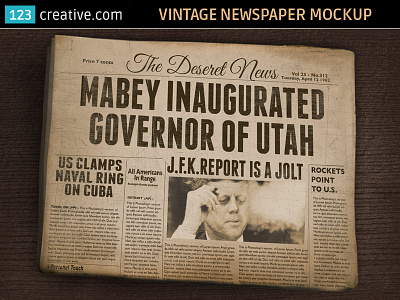The image depicts a vintage replica of a folded newspaper called "The Desert News" with a black background, showcasing the upper half of its front page. Dominating the headlines is "Maybe Inaugurated Governor of Utah," alongside a significant headline reading "JFK Report is a Jolt" accompanied by a photograph of John F. Kennedy, signifying it's from the early 1960s when Kennedy was still alive. On the left side, there's a headline that states "U.S. Clamps Naval Ring on Cuba," indicating the era of the Cuban Missile Crisis. Another smaller headline reads "Rockets Point to US." The reproduction is identified at the top of the image by "123creative.com" in a blue rectangle with white lettering, and "Vintage Newspaper Mock-Up" in tan lettering on the right corner, suggesting that this is a creative depiction rather than an actual newspaper. The newspaper is considerably aged, with a discolored and antique appearance, further reinforcing its vintage look.